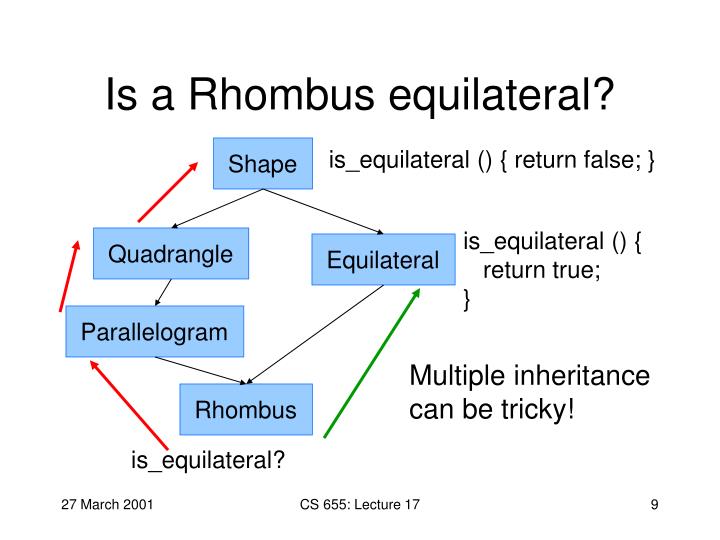The image depicts a slide from a presentation, titled "Is a Rhombus Equilateral?" in black text at the top. Below the title, there is a flowchart consisting of blue rectangular boxes with labels written in black text. The first box at the top is labeled "Shape," followed by sequential boxes labeled "Quadrangle," "Parallelogram," and "Rhombus." To the right of these, there is a box labeled "Equilateral." Arrows in green, red, and black point from one box to another, illustrating relationships or questions about equilateral properties. The diagram includes logical statements like "is equilateral return false" and "is equilateral return true," as well as a note stating "multiple inheritance can be tricky." The bottom left-hand corner of the slide displays the date "27 March 2001" and mentions "CS 655 lecture 17" in a different font. The overall arrangement of arrows and text appears a bit complex and might require further explanation for clarity.